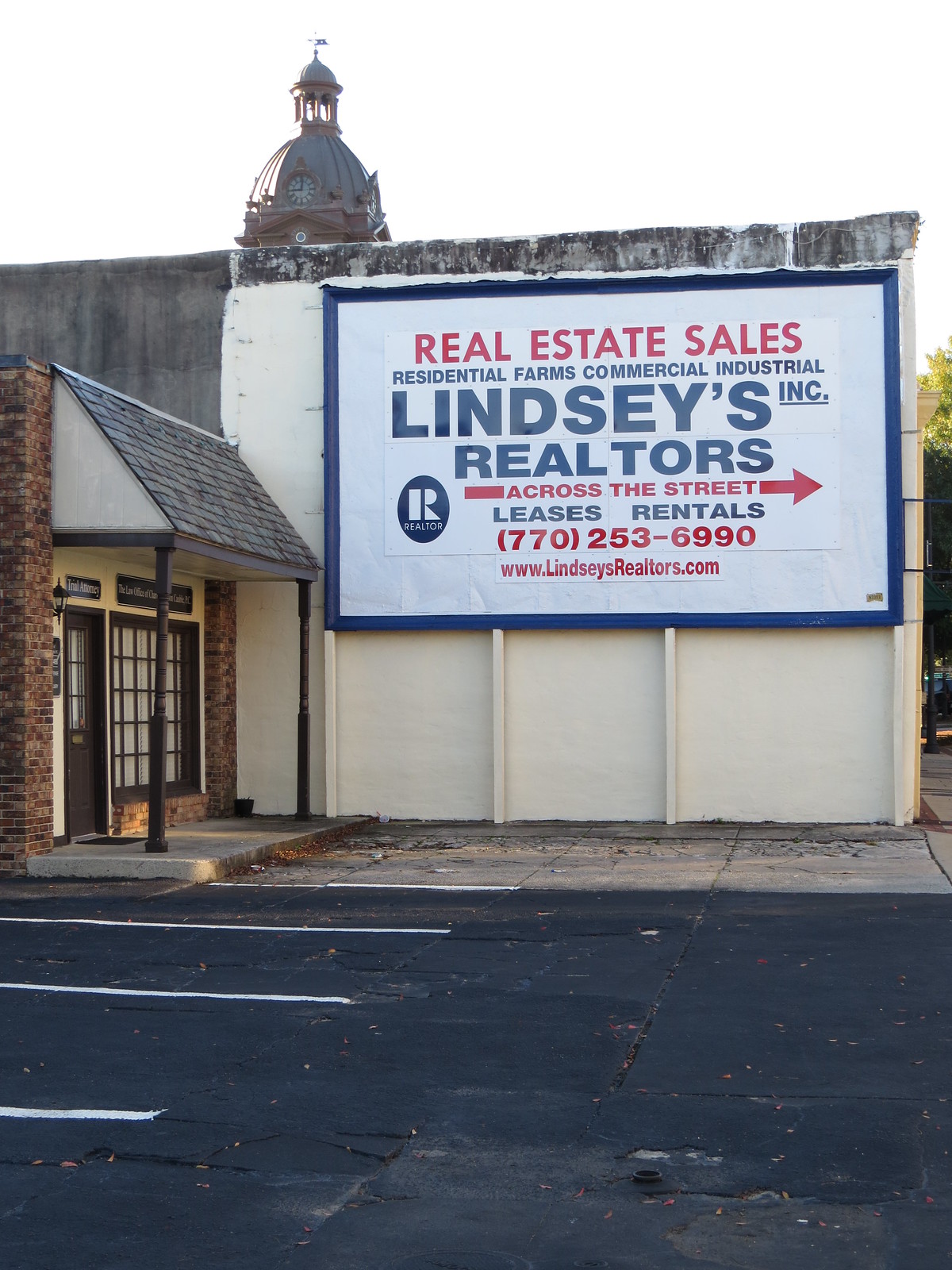The photograph captures a somewhat dilapidated one-story building with a brown wooden door and brown wooden-framed windows, both bordered by red bricks. A portico with a small roof overhangs the entrance. The structure is situated in a neglected parking lot, characterized by several cracks and an overall unkempt appearance. At the forefront, a large, blue-framed sign with a white background prominently displays: "Real Estate Sales" in red, while below it, in blue text, it lists "Residential Farms, Commercial Industrial, Lindsay's Inc., Realtors". An arrow in red points to the right with the words "Across the Street", and below that, further information in blue reads "Leases, Rentals", along with a phone number, 770-253-6990, and the website www.lindsayrealtors.com. In the distant background, the top of a stately building is visible, featuring a domed roof, a clock, and a small flag atop it, which resembles a government building or a clock tower. The clock indicates an approximate time of nine o'clock in the morning.